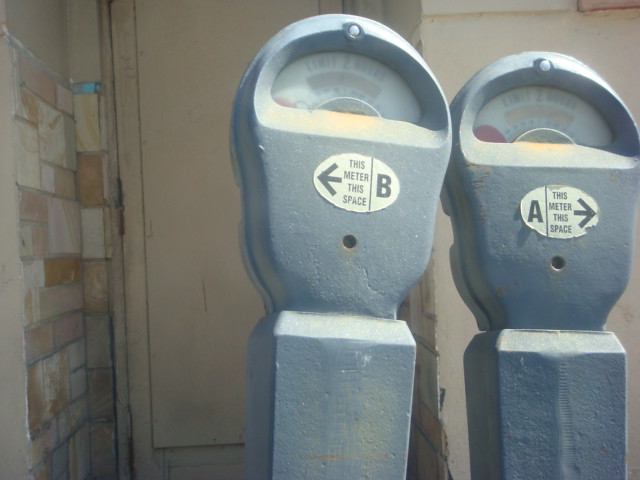The photograph showcases two old, rusted parking meters leaning against each other, suggesting they might be out of use or set aside in an entryway or alley. Each meter features a distinct rounded top, resembling a thumb, transitioning into a rectangular body. At the top of the meters, there are opaque plastic or glass screens, through which the faded and cloudy text can be barely discerned. Below the screens, stickers labeled "This Meter, This Space" point in different directions: the left meter labeled 'B' points left, and the right meter labeled 'A' points right, with a limit of two hours indicated for parking.

The environment around the meters includes a textured brick hallway and a tile base that wraps around to the right, where it meets a white wall. A tan, wooden door stands behind the meters. The details of the surroundings, such as the brick and white tiling, add depth to the setting, highlighting the aged and possibly abandoned nature of the scene.